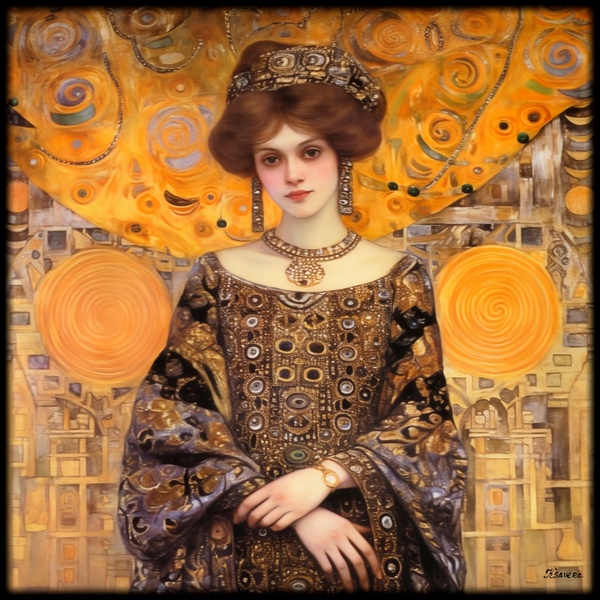This large, square oil on canvas painting, enclosed in a thin black frame with a subtle shadow effect at the border, features a portrait of a melancholic young woman, seemingly in her late teens, with milky white skin and subtly rosy cheeks. Signed by the artist "SAVERA" in the lower right corner, the artwork captures the woman from just below the waist up, highlighting her intricately styled brown hair, swept to the sides and pulled back into an updo adorned with a gold headdress. Her neutral expression is softened by her large brown eyes, and she wears long, dangling rectangular earrings that complement her elaborate, jeweled necklace with a prominent pendant. The woman's Victorian-style dress, characterized by its off-the-shoulder design and long, flowing, baggy sleeves, features a brown fabric embellished with gold and black accents. On her left wrist, she sports a thin gold watch. The background is a harmonious blend of lighter shades of her dress's colors, adorned with abstract circular and geometric designs in yellow, gold, and tan, including two prominent swirling patterns resembling the tops of lollipops, and a larger circle descending from the top, punctuated with smaller spirals and squares.